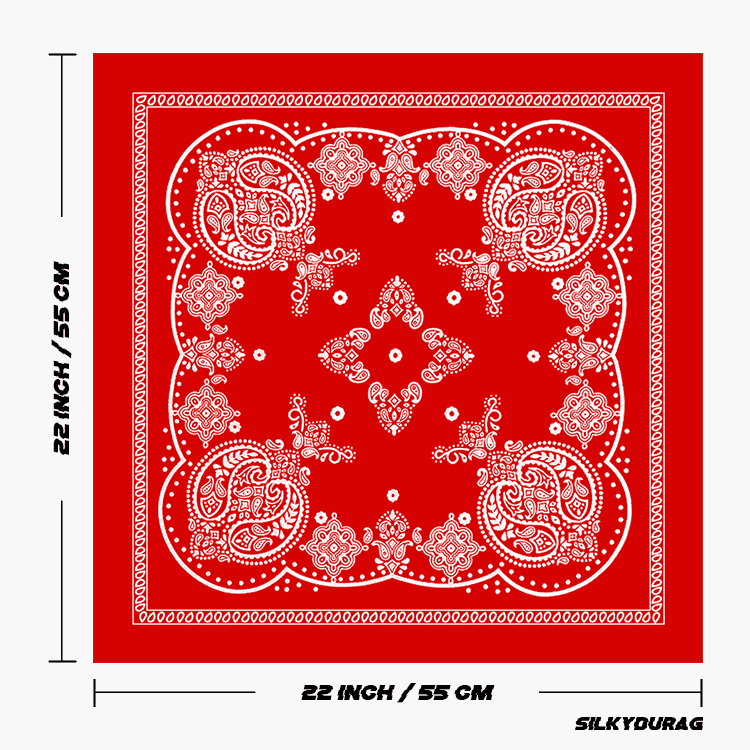The image depicts a red silk bandana (also referred to as a do-rag) which measures 22 inches by 22 inches (55 centimeters by 55 centimeters). The bandana features intricate white designs that give it a paisley-like and slightly bohemian appearance. The fabric is adorned with a symmetrical, ornate pattern consisting of various shapes such as teardrops, circles, and squares.

The border of the bandana is square-shaped and is lined with small, white, oblong circles that create a delicate edging around the perimeter. Inside this border is another rectangular border, approximately one inch inside from the edge, also decorated with tiny white circles. This inner border frames the central design, which is structured around a diamond-shaped pattern filled with elaborate, wavy lines and curls resembling the traditional Scottish Paisley pattern.

At each of the four corners of the bandana, the design features larger decorative elements that mirror one another, enhancing the symmetry of the entire piece. The background of the fabric is red while all the decorative elements are in white, creating a striking contrast.

Measurement annotations are present on the left side and the bottom of the image, both indicating "22 inch / 55 centimeter." Additionally, in the bottom right corner, the text "Silk Silky Do-Rag" is displayed, confirming the stylish and silky nature of the fabric.